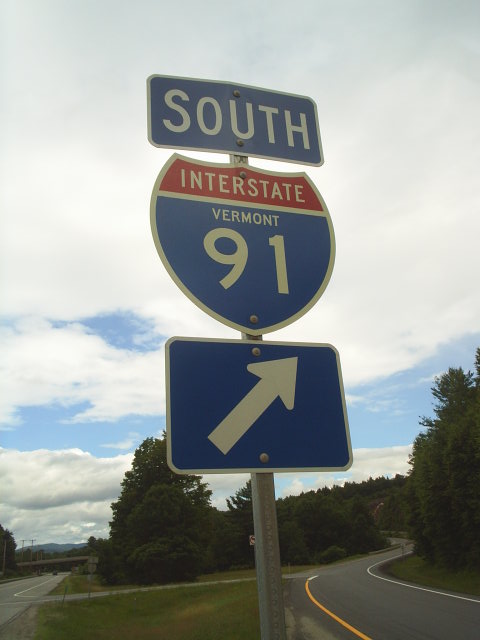This detailed photograph features a prominent highway sign centered in the image. The sign is composed of multiple components: the top segment is a blue rectangle displaying the word "South" in white text, enclosed within a metallic border. Directly below, a distinctively shield-shaped symbol prominently marks this route as "Interstate Vermont 91," with the word "Interstate" appearing in white text against a red background at the top of the shield. Beneath the shield is another blue sign in a rectangular shape, showcasing a white arrow pointing diagonally to the right.

The background adds context to the sign's location. On the left side, there is a visible highway, while another highway on the right curves gently and leads into a dense row of trees. This side of the image features a significant expanse of trees. The sky is a mix of blue with a considerable number of clouds, some of which appear to be darkening towards the horizon, possibly indicating an impending storm. This intricately captures not only the highway sign but also the surrounding environment, providing a comprehensive view of the scene.